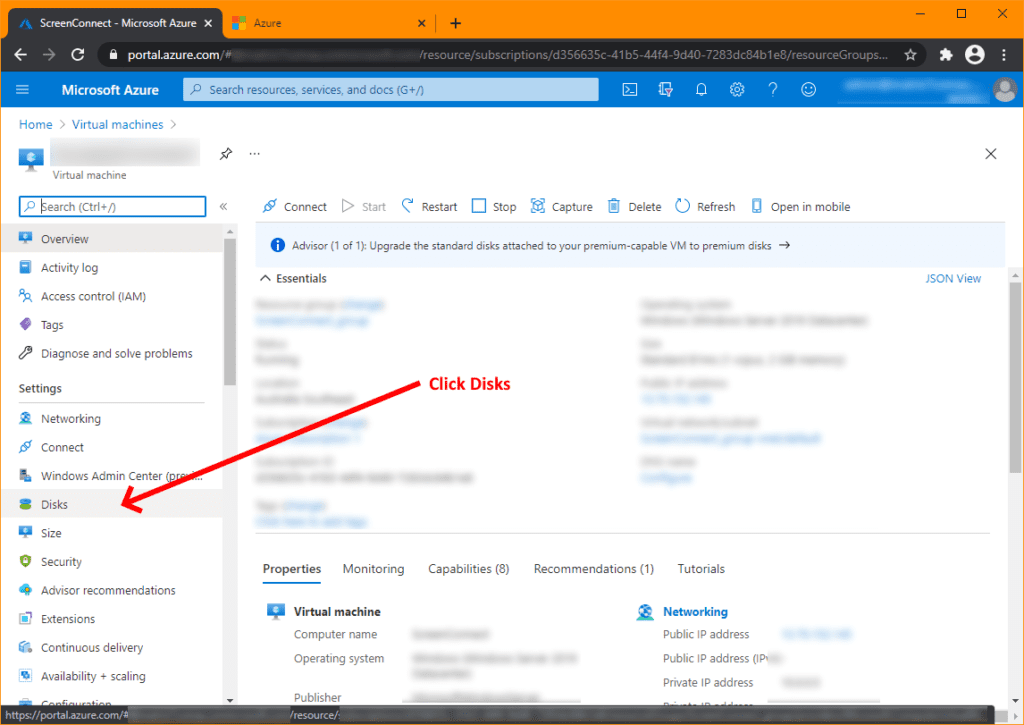The image depicts a computer screenshot with two open browser tabs in incognito mode, as indicated by the dark gray search bar. The first tab is labeled "Screen Connect," featuring a blue logo on the left, while the second tab is titled "Azure," displaying the well-known Microsoft logo composed of red, green, yellow, and blue squares.

Currently, the screen is focused on the "Screen Connect Microsoft Azure" tab. The webpage is highlighted by a blue banner displaying the Microsoft Azure logo. Positioned on the far right, the top bar includes a search bar, and an icon photo beside various interactive icons, such as notifications, settings, and a help section. The user's personal name or account information appears next to the icon photo but is blurred for privacy.

The primary content of the webpage pertains to the management of virtual machines. Below the banner, there is a navigation path indicating the user is exploring options under "Home > Virtual Machines." The left sidebar contains a search bar and multiple clickable options, with a prominent red arrow pointing to the "Disks" settings, accompanied by a note reading "Click Disk," directing the user to select this particular option.

The main section, to the right of the sidebar, shows an "Essentials" segment, but most of its text is obscured. At the bottom of this section, a detailed menu provides further options, including "Properties," "Monitoring," "Capabilities," "Recommendations," and "Tutorials." On the left side of this essentials area, there's an icon for virtual machines, and on the right, an icon for networking completes the available options.